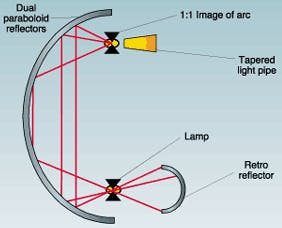The image is a diagram of a light electronic device featuring various components and directional indicators. On the upper left corner, the text reads "dual paraboloid reflectors." The central part of the diagram showcases a large C-shaped arc, with several red lines illustrating the path of light. At both the top and bottom ends of the C-shape are identical black bow-tie-like objects. The text next to the upper black object indicates "1 to 1 image of arc," while an attached shape resembling a cup or a cone is labeled "tapered light pipe," signifying the direction of light towards a convex surface on the left. The lower black object, accompanied by the text "lamp," similarly directs light through the apparatus. Below the main C-shape, an inverted smaller C is labeled "retroreflector." The overall design emphasizes the structured reflection and redirection of light through the specified components.